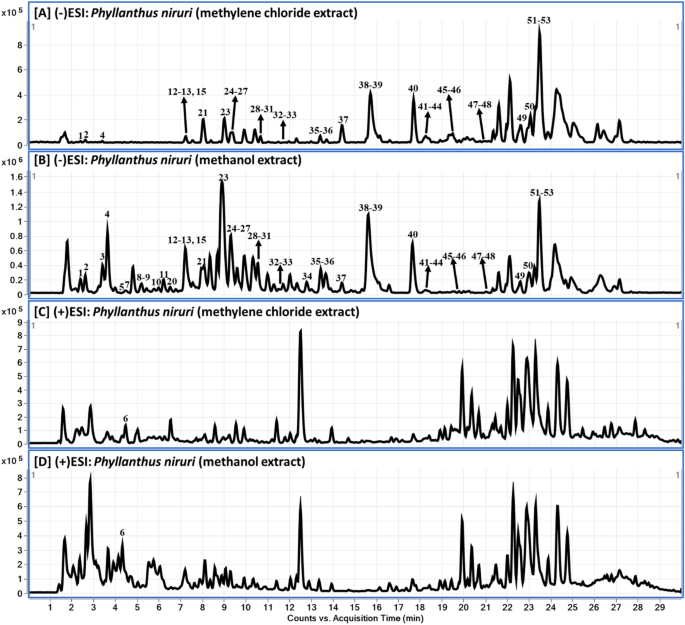This image depicts four vertically stacked graphs labeled A, B, C, and D, each associated with a scientific experiment or study involving chemical extracts. The common x-axis of these graphs is labeled "Counts vs. Acquisition Time Minutes," spanning from 1 to 29. Each graph features an EKG-like pattern with lines oscillating up and down, indicating varying data points. 

For the y-axis:
- Graph A represents "Fulfanzas Neri Methylene Chloride Extract" and ranges from 0 to 10.5.
- Graph B shows "Fulfanzas Neri Methanol Extract" with a similar scale.
- Graph C, like Graph A, displays "Methylene Chloride Extract" ranging from 0 to 10.5.
- Graph D, akin to Graph B, indicates "Methanol Extract" with the identical range.

The numerical data and the complex scientific terminology, appearing in both Latin and English, suggest the graphs detail the results of a detailed chromatographic analysis, each extract exhibiting distinct peaks and valleys indicative of their unique chemical signatures.